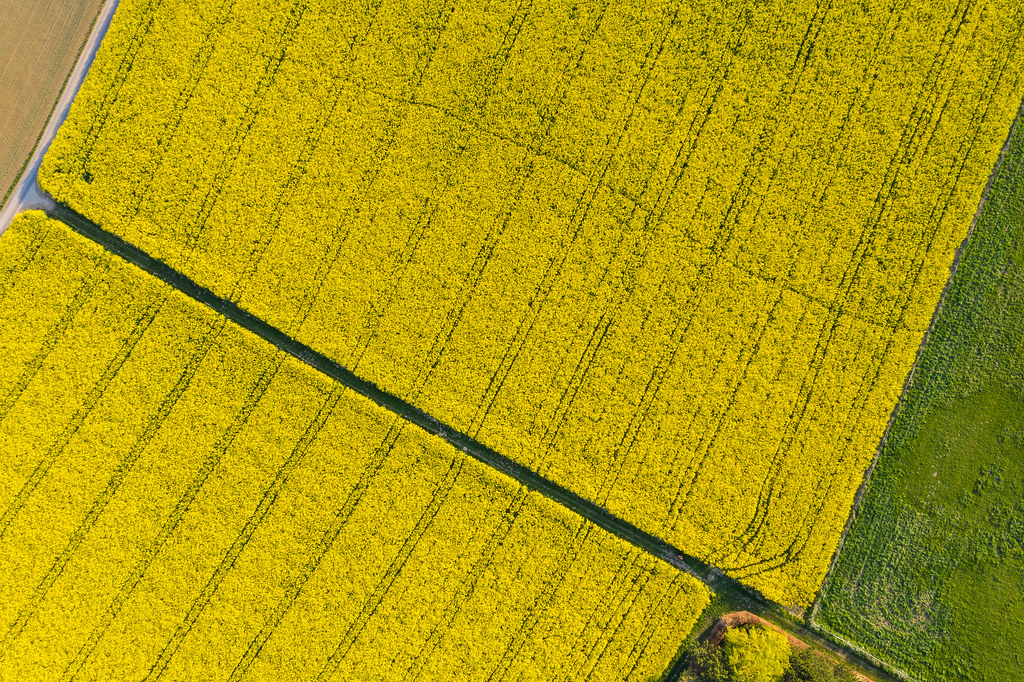This aerial photograph provides a captivating overhead view of meticulously tilled fields, likely captured from a drone or helicopter. The landscape is predominantly composed of rectangular sections of light yellow-green plants that appear uniformly planted in neat rows. These fields are divided by green lines, indicative of pathways or small roads. The upper left corner of the image transitions into a sandy tan area, while the upper and most of the right side showcases the bright yellow-green fields. In contrast, the bottom right corner features a darker green triangular patch of grass. This grassy section stands out with a vibrant hue against the lighter fields. Midway through the image, separating the yellow-green fields, appears to be a dirt road or pathway. Additionally, a small triangle of light yellow and green plants can be seen at the bottom. The scene is devoid of any human presence, equipment, or buildings, creating a serene agricultural tableau focused solely on the cultivated land and its inherent patterns.